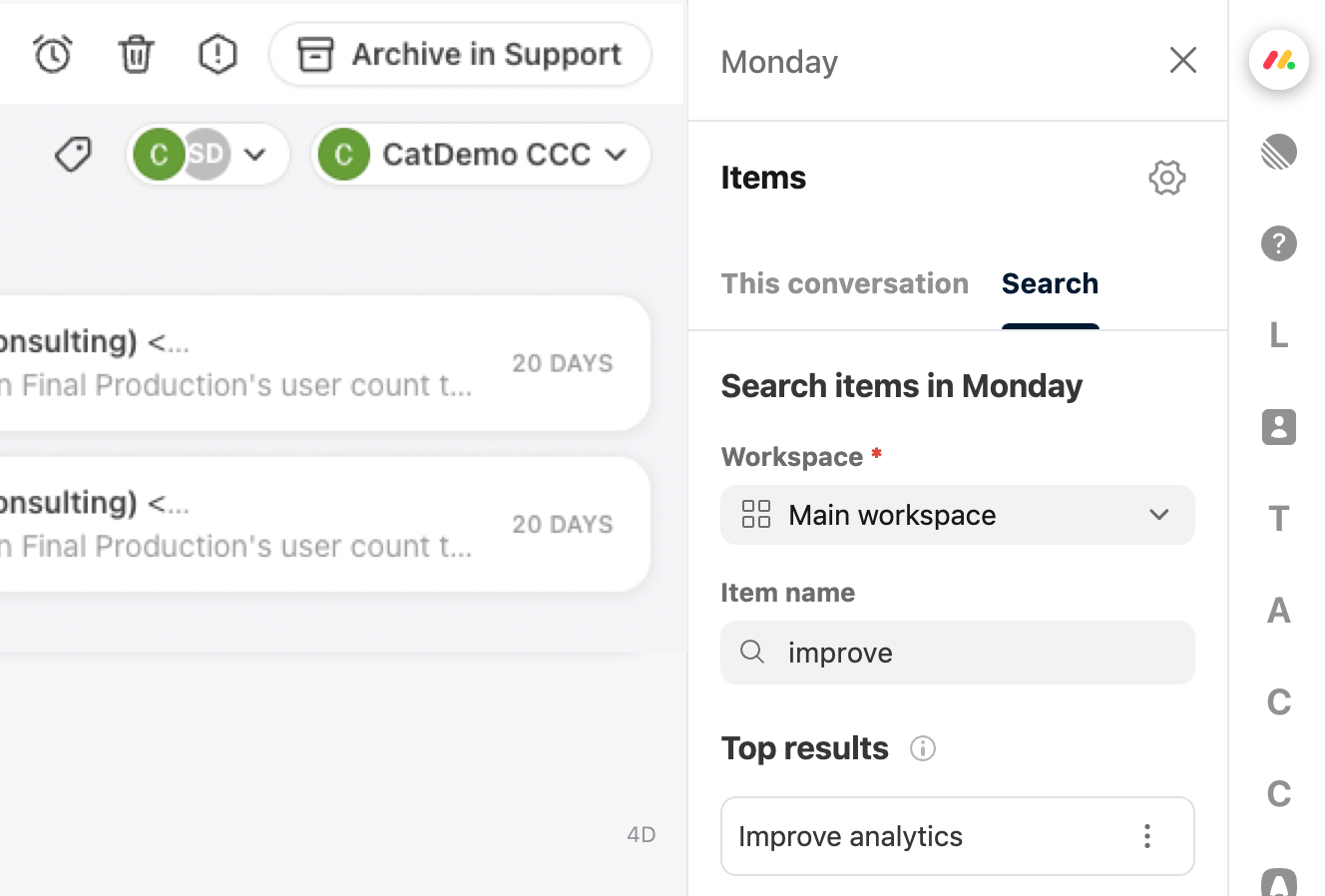This rectangular image is oriented with its longer sides extending horizontally. On the left-hand side, the image features a vertical column hosting a variety of icons and labels. At the top of this column, there is an alarm clock icon, followed by a garbage can icon, a hexagonal shape, and an open box labeled "Archive in Support." 

Below these icons, there is a gray box with the label "Cat Demo" at the top that appears to contain several posts or pieces of information, although the text is somewhat hard to read. Phrases like "Final Productions," "User Count," and "20 Days" are faintly visible, suggesting it's related to user statistics or project timelines.

As we move towards the right side of the image, another column emerges. This column has "Monday" written at the top, accompanied by an 'X' icon on the right, likely indicating a close or delete option. The column starts with a thin gray line that separates it from the next section labeled "Items." Below this, a bold 'Search' text is visible, indicating a search function within "Items." This is further divided by another thin gray line.

Moving down the column, there's a label "Search Items in Monday," followed by "Workspace, Main Workspace, Item Name," and a section labeled "Improve," which includes the top search results for "Improve Analytics."

On the far right of this layout, a vertical strip runs from the top to the bottom of the image. This strip contains a series of icons and letters, including 'L,' 'T,' 'A,' 'C,' and 'C,' running vertically. Additionally, there is a person icon and a question mark icon within this strip, possibly representing user settings and help features, respectively.